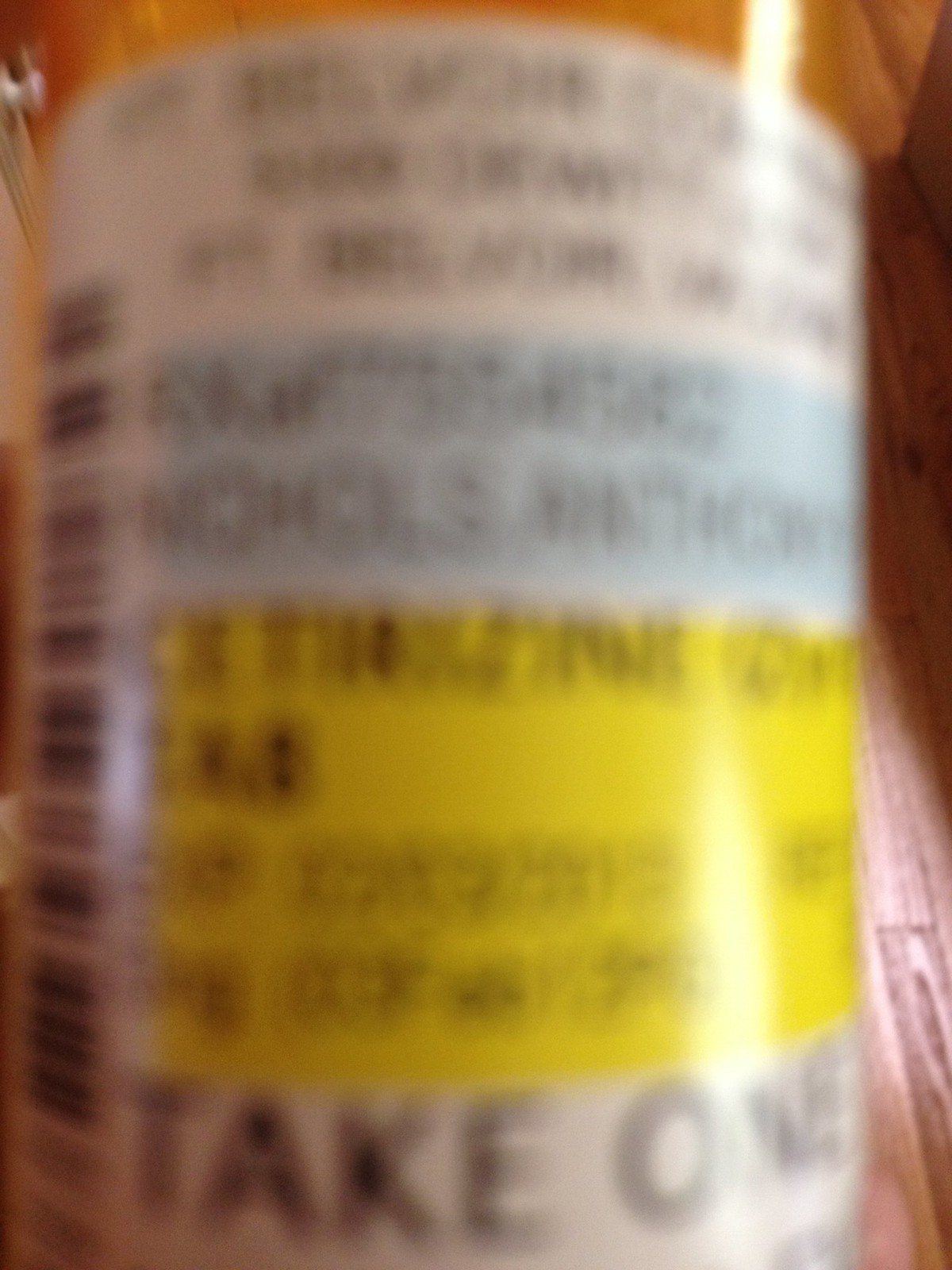The image depicts a close-up of a prescription bottle, characterized by its signature cylindrical shape and amber-brown color. The bottle's label is predominantly white with blue and yellow accents, though the specific details are obscured due to significant blurring. A vertical barcode is visible along the left-hand side of the label. In the clearer, white section at the bottom of the label, the text "take one" can be discerned, indicating the prescribed dosage.